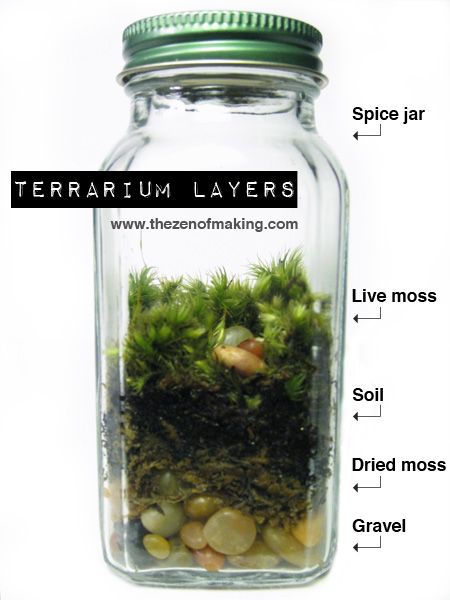The photograph is a detailed instructional image demonstrating how to create a terrarium in a square-edged, milk carton-style glass jar with a rounded top. At the bottom of the jar, there is a layer of gravel, followed by a layer of dried moss soil, and then a layer of live moss that appears to be thriving. Each layer is labeled with black text and arrows: "Gravel" at the bottom, "Dried Moss Soil" in the middle, and "Live Moss" at the top. The jar is described as a "Spice Jar" in a black arrow pointing from the top right. Above the photograph, a strip of white typewriter-style font on a black background reads "Terrarium Layers." At the middle of the jar, the website "www.thezenofmaking.com" is displayed in gray font. The jar is sealed with a green lid, completing the informative and visually appealing depiction of the terrarium's construction.